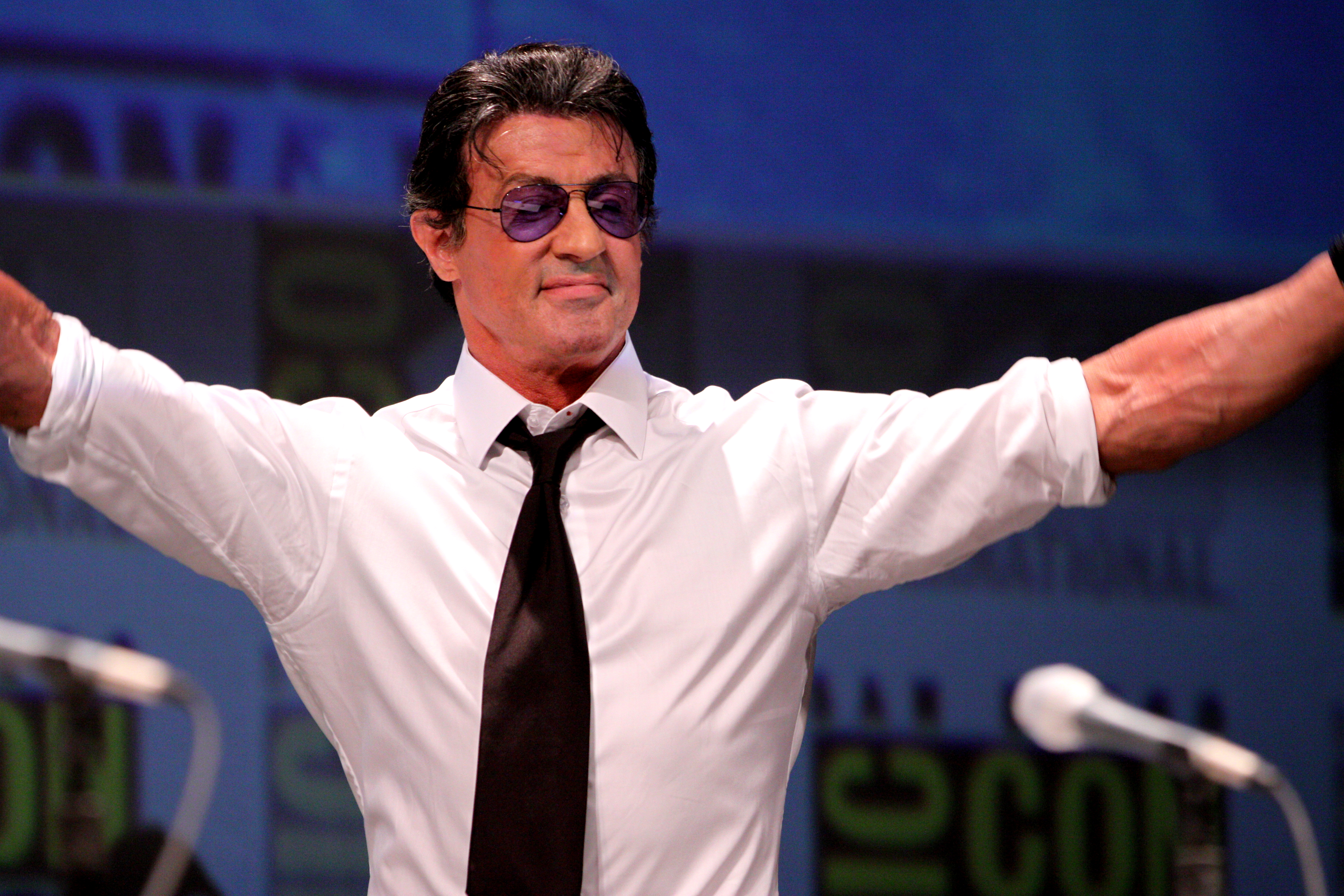The horizontally aligned photograph captures Sylvester Stallone, the actor famed for playing Rocky Balboa, standing slightly to the left of center on stage at what appears to be Comic-Con in San Diego. The blue backdrop is adorned with repeating San Diego Comic-Con logos in yellow, black, green, and some faded letters. Stallone's slicked back, short black hair frames his tan, clean-shaven face, which is accented by purple, somewhat oval sunglasses. He is dressed in a long-sleeved white collared shirt with the sleeves rolled up past his elbows, exposing his veiny arms. A slightly loosened black tie hangs around his neck. Smiling with his lips pressed together, he spreads his arms wide in a gesture that conveys a sense of pride. In front of him, two silver microphones attached to black stands are positioned in the lower corners of the image. The overall atmosphere suggests a recent decade, likely the 2000s, capturing Stallone engaged with his fans at a speaking event.